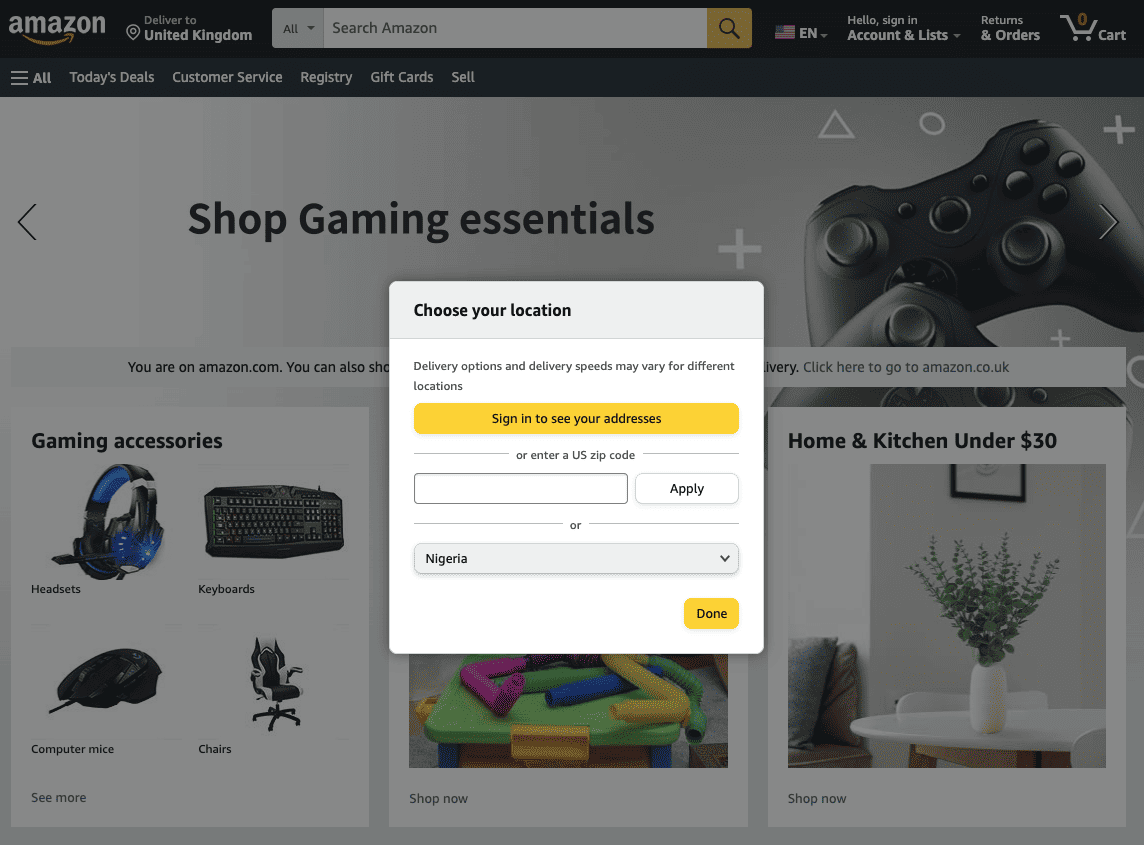This is a screenshot captured in landscape mode, likely from a laptop, displaying an Amazon shopping page focused on gaming essentials. The top part of the image features a black stripe background spanning from the upper left-hand corner to the upper right-hand corner. In the upper left-hand corner, the Amazon logo is prominently displayed, followed by the text "Deliver to United Kingdom" with a location icon.

Next to this is the search bar, set to query all of Amazon, and adjacent to the search bar is the American English flag. Further right, the page reads "Hello, Sign in," followed by "Accounts & Lists," "Returns & Orders," and a cart icon showing zero items.

Beneath this primary navigation bar, there is a dark gray stripe extending from left to right, featuring options like "Today's Deals," "Customer Service," "Registry," "Gift Cards," and "Sell."

Below this stripe, a large image promotes gaming essentials, accompanied by a pop-up message prompting the user to "Choose your location." This message appears on a semi-transparent gray background, stating that delivery options and speeds vary by location. It includes a form with a large orange "Sign in to see your address" button, or allows users to enter a US zip code. The form contains a clear "Apply" button on the right.

Additionally, there is a default selection for "Nigeria" in a drop-down menu with an arrow. The bottom right-hand corner of the pop-up features an orange "Done" button.

The remainder of the page showcases various gaming accessories, and in the right-hand section, additional categories like "Home and Kitchen under $30" are visible.